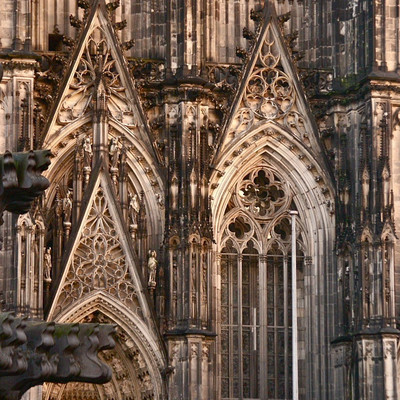The image depicts the intricately designed facade of a majestic, old cathedral, resembling the architectural splendor of renowned churches such as Notre Dame in Paris. The structure prominently features two detailed, large, arched doorways, the surfaces of which exhibit a grated design, complemented by singular cylinder door handles. Above each doorway is a triangular inset adorned with elaborate ornamentation, showcasing superior craftsmanship and intricate motifs. The cathedral, primarily composed of off-white, brown, and gray hues, exudes an ancient, timeless beauty. Flanking these central doorways are additional triangular insets, with one on the left side featuring a light above it. The architecture includes tall, peaked arches and visible crosses embedded within the design, suggesting a Renaissance Byzantine style characterized by both height and intricacy. The upper parts of the structure, glimpsed at the top edges of the image, hint at towering spires, potentially stretching over 100 feet high. Gargoyles, though out of focus, are discernible in the foreground, adding to the overall grandeur and historical significance of this monumental cathedral.